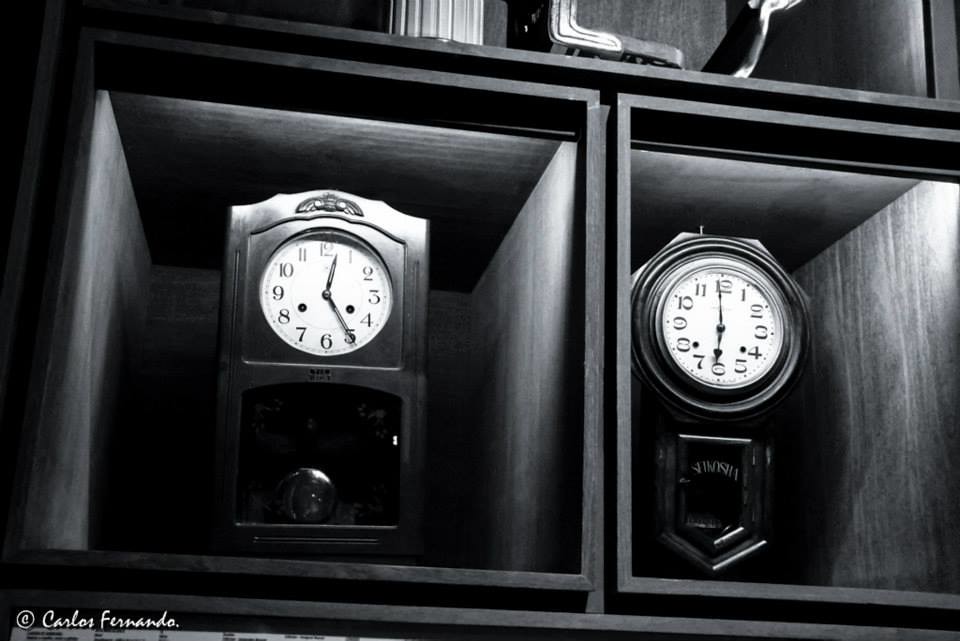Photographed by Carlos Fernando (© Carlos Fernando), this detailed image captures a charming display of two pendulum clocks arranged within a dark wooden box. Each clock is snugly positioned in its own cubby made of rich, dark-stained wood, emphasizing their timeless appeal. The clocks themselves are crafted from wood and feature elegant, swinging pendulums visible through small, glass-windowed doors. The faces of the clocks are adorned with Arabic numerals, adding a classic touch to their vintage design. The setting appears to be a part of a larger display, possibly in an antique or second-hand store, as suggested by the partially visible objects placed on the shelf above, which are not clocks. This carefully curated scene suggests a possible invitation for potential buyers or offers a glimpse into a collector's treasured assemblage.